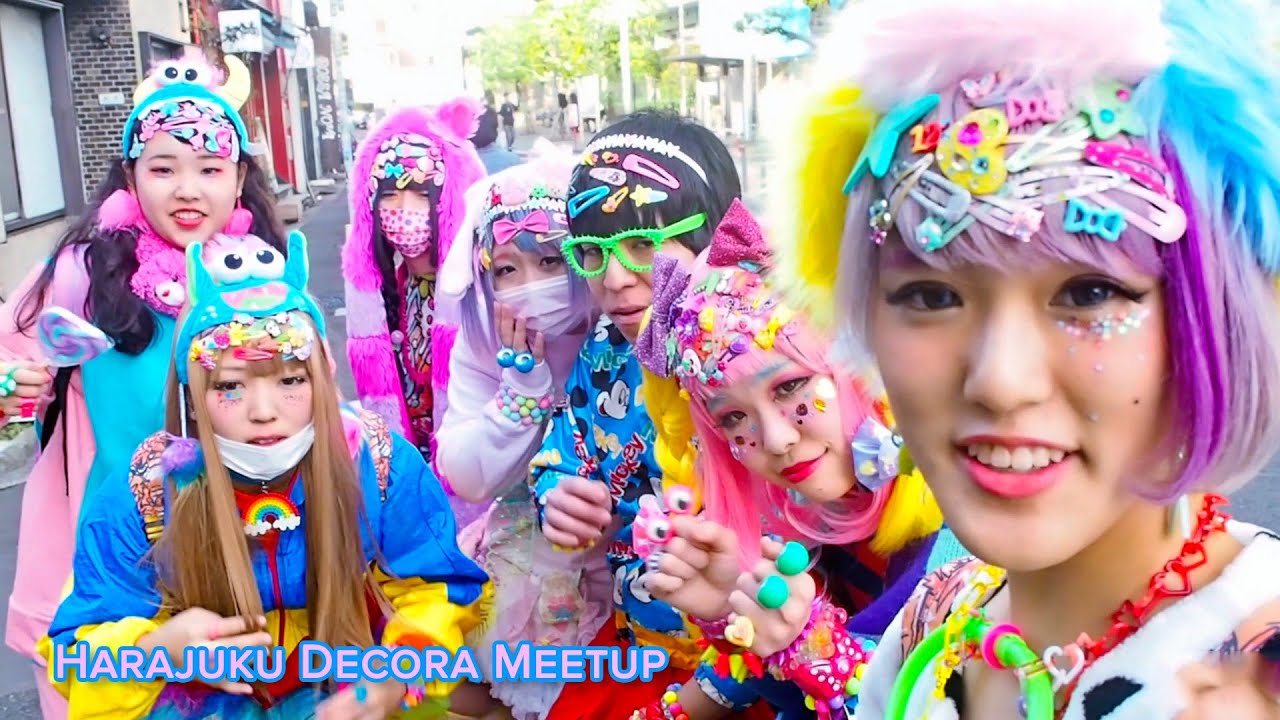In a vibrant display of Harajuku Decora fashion, the image features a group of six women and one man, each adorned in bright, childlike costumes and colorful accessories. The women are wearing vivid wigs and headpieces fashioned as fuzzy cartoon characters with large, expressive eyes, some of which are reminiscent of Cookie Monster's head with eyeballs. The costumes incorporate primary shades of purple, pink, and blue, adding to the lively palette. The scene is set outdoors against a backdrop of a bustling cityscape with tree-lined streets and various shops. The man, distinguishing himself with black hair and green glasses, is positioned centrally in the group. Several members of the group are wearing makeup, and some of the women have masks covering their noses and mouths while others do not. At the bottom left of the image, in purple text trimmed in blue, the caption reads "Harajuku Decora Meetup." The photograph, capturing this eclectic and colorful assembly, seems poised as a potential social media post, possibly to attract influencers or announce the meetup in the famous shopping area of Japan’s Harajuku district.